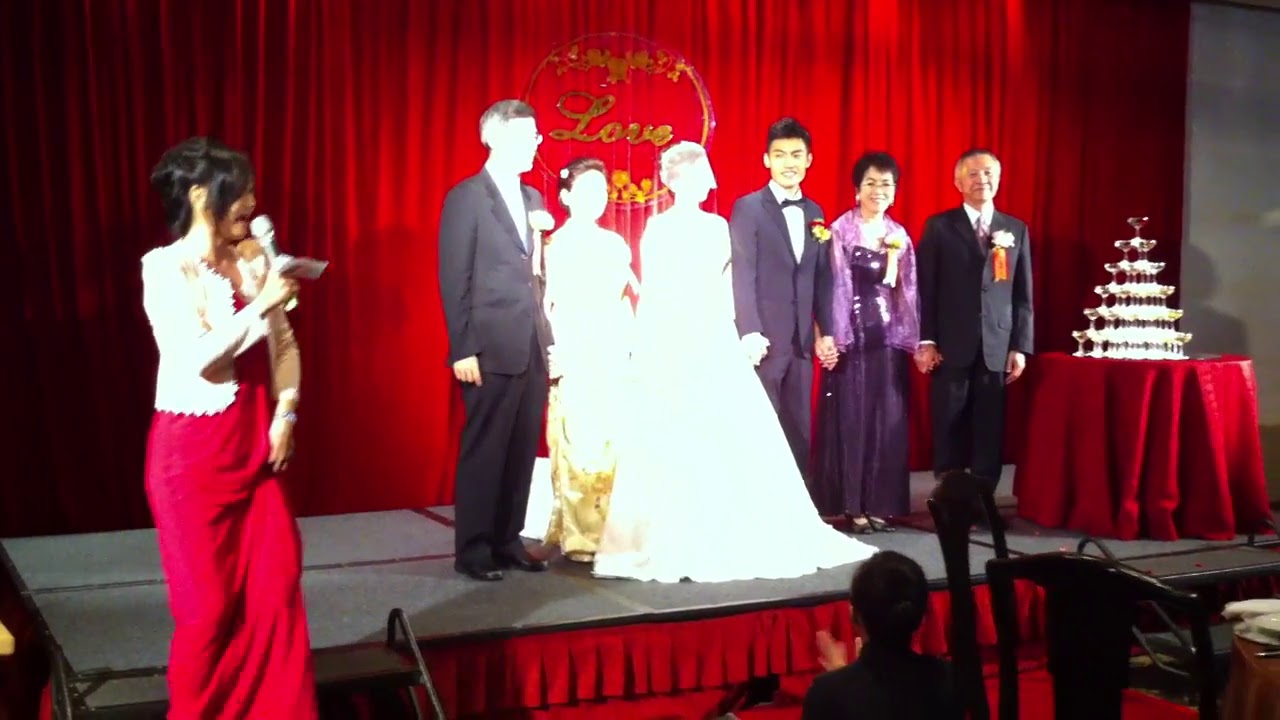In this image, we see a wedding scene with a group of six people standing on a small stage adorned with bright red curtains and a golden sign that spells "LOVE," set against a backdrop of pink and yellow flowers. On the left side of the stage, a woman in a red dress with a white bolero is speaking into a silver microphone. Behind her, another woman, possibly the bride, is dressed in a flowing white gown, standing next to an older woman in a white dress, likely her mother. To the bride's left stands a man in a suit, possibly her father, whose face is somewhat obscured by intense glare, making it difficult to discern details. To the right of the bride, we find the groom, dressed in a black or gray suit with a flower in his pocket, accompanied by his parents—his mother in a purple gown with a matching shawl and a yellow flower on her chest, and his father also in a suit. Positioned to the right of the stage is a striking pyramid of champagne glasses sitting atop a table draped in a red tablecloth. Just below the stage, at the foot of the stairs, an individual appears to be clapping, while dark railings and black equipment frame the scene, contributing to the festive indoor setting.